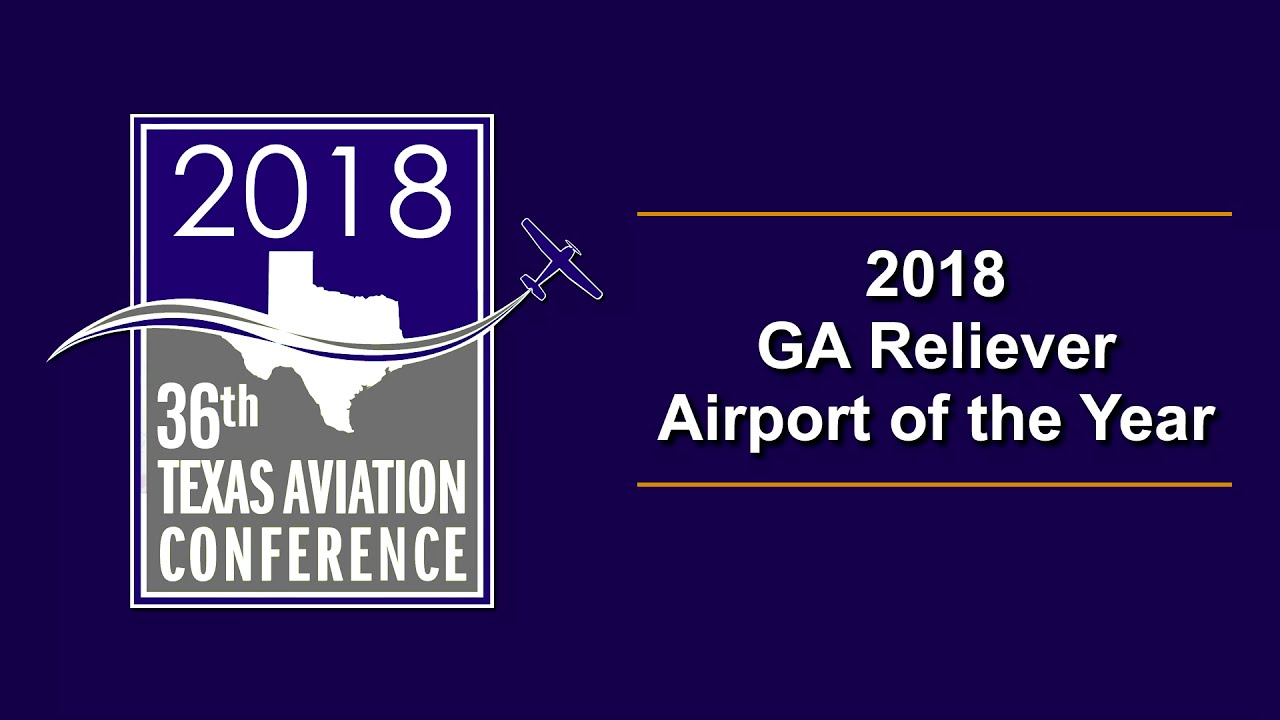The image is a banner advertisement with a primarily dark navy blue background, transitioning to a lighter purplish hue towards the bottom. On the left side, there's a rectangular logo divided into an upper navy blue section and a lower gray section. The top part of the logo features the year "2018" in white text, while the bottom part prominently displays "36th Texas Aviation Conference" also in white. The logo is detailed with multiple borders: a white border, followed by a blue outline, and then another white outline. A small, blue single-prop airplane with a white outline flies from the left side of the logo, leaving a wavy smoke trail that separates the blue and gray sections and extends outside the logo box.

The right side of the banner is bordered by gold lines at the top and bottom. Between these lines, in bold white text, it reads "2018 GA Reliever Airport of the Year." The entire composition of the banner emphasizes the Texas state silhouette in white, highlighted by the airplane’s smoke trail crossing through it, symbolizing the aviation theme and the conference's significance in Texas.